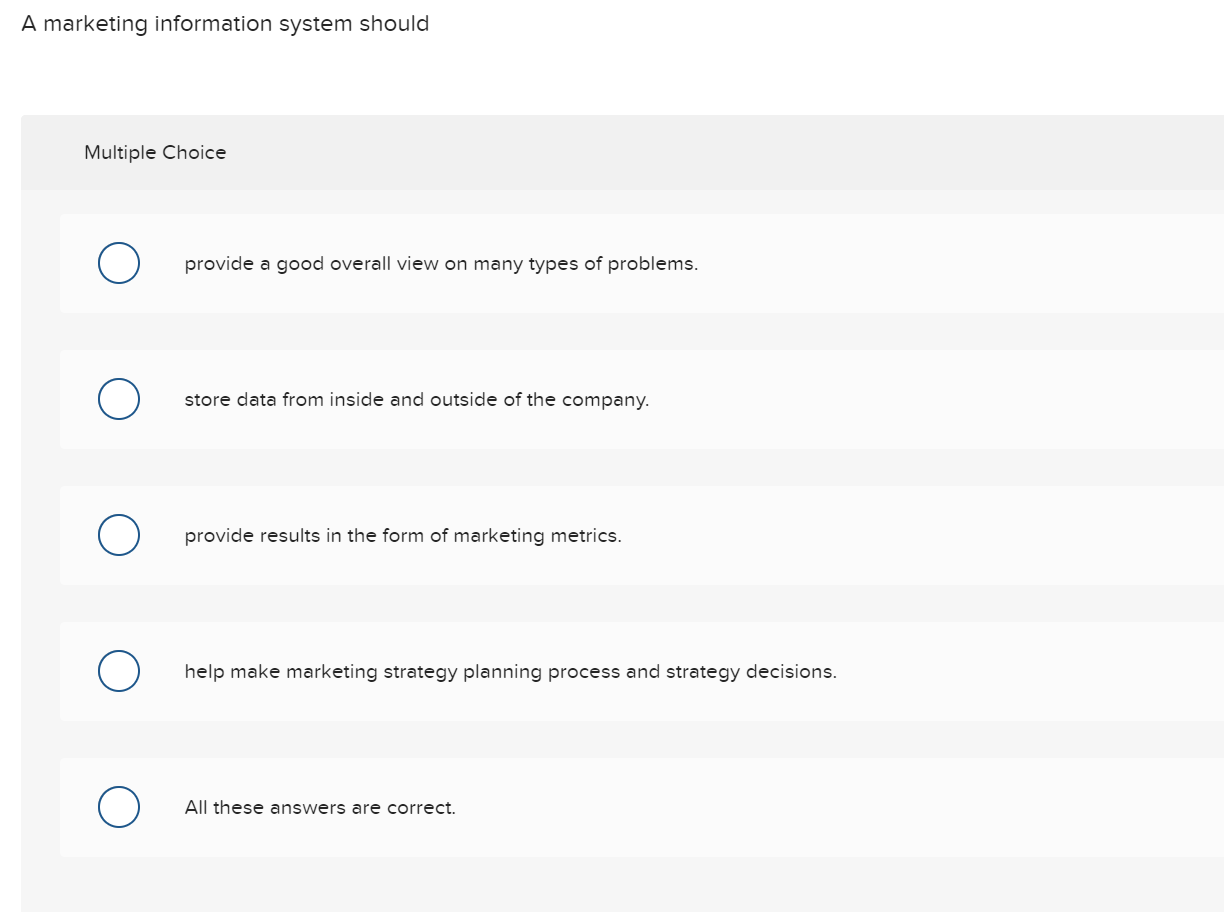This image displays a multiple-choice question from an electronic test on someone's computer screen. The interface has a clean and structured layout with a white border at the top containing the black text of the question. The question reads: "A marketing information system should:"

Below the question is a gray section labeled "Multiple Choice" on the left side. Within this gray area, five answer options are listed, each preceded by a blank circle. The options, set against a white background, are as follows:

1. Provide a good overall view of many types of problems.
2. Store data from inside and outside of the company.
3. Provide results in the form of marketing metrics.
4. Help make marketing strategy planning processes and strategy decisions.
5. All these answers are correct.

The layout includes gray borders on the left and right sides, as well as at the bottom of the screen. The image is strictly textual with no pictures or human figures, focusing solely on the black text against the gray and white background for a clear and uncluttered presentation.